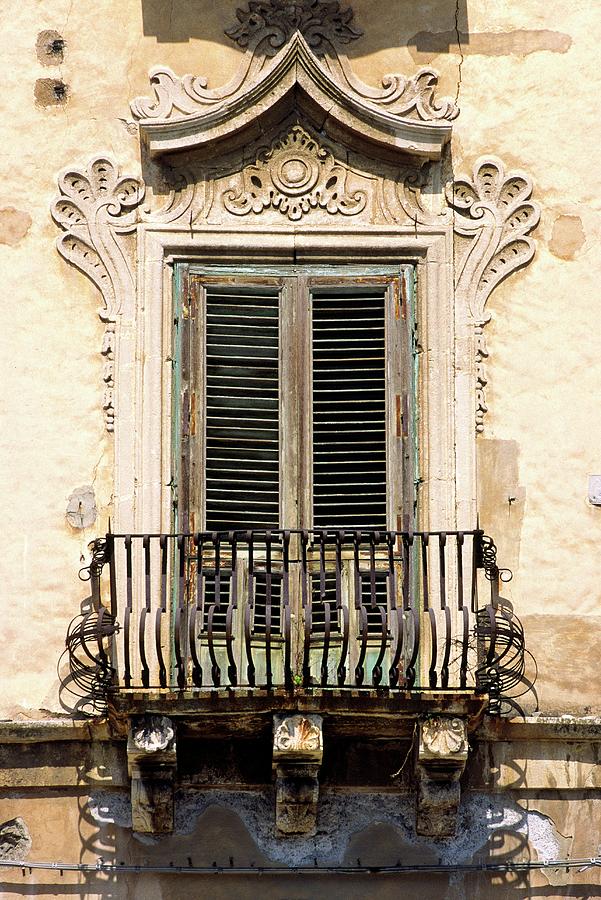This outdoor photograph features a rustic, 18th-century-style balcony on a beige-toned building. The balcony, modestly sized at about 6 feet wide, is framed by a set of brown, weathered wooden double doors that double as shutters, showing signs of age with chipping paint and worn wood strips. These doors are set within a detailed stone frame, complete with stylized molding and an elaborate inverted V-shaped roof that has some floral motifs on either side. Iron elements, shaped into bold, swirling designs, form the wrought iron railing of the balcony, which appears somewhat dilapidated and darkened by age. This railing is supported by three stone beams underneath, which show signs of wear and cracking, adding to the overall historic and slightly neglected aesthetic of the scene.